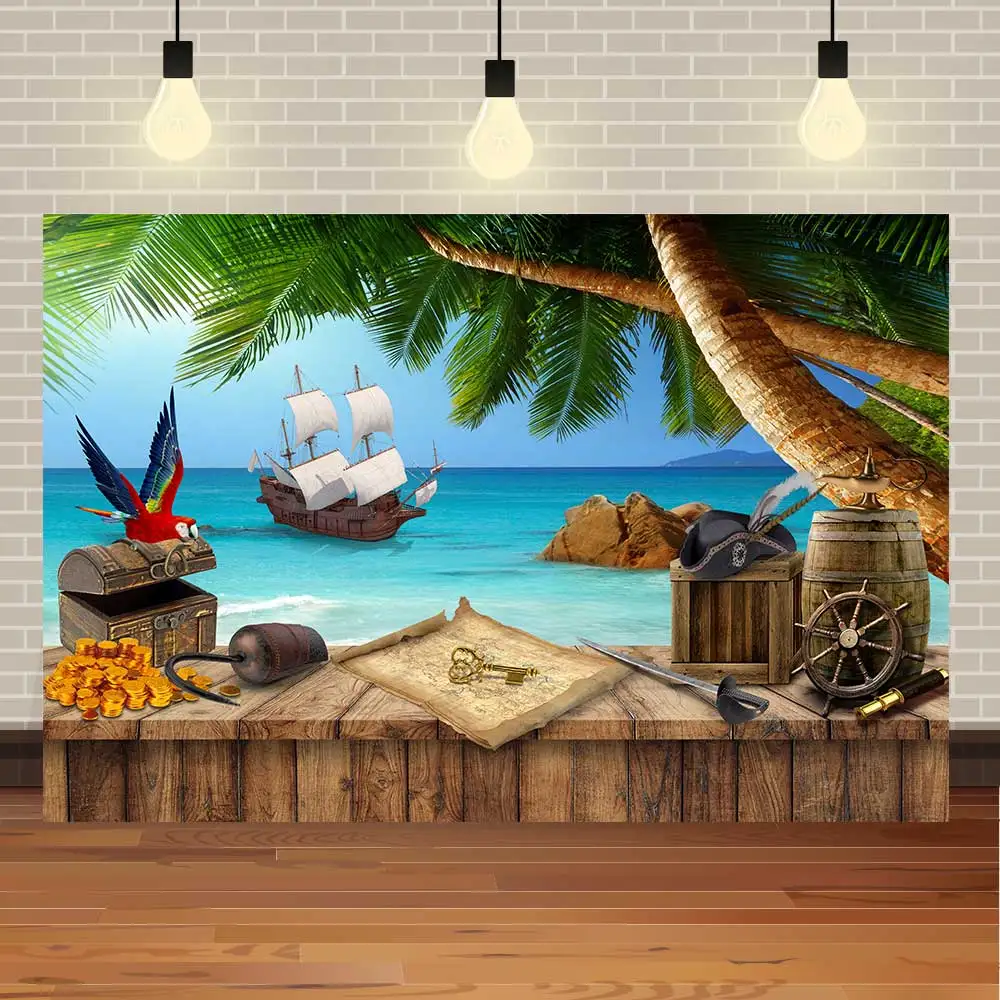The image portrays an intricately detailed and almost three-dimensional painting of a seaside setting, featuring a vibrant mix of pirate-themed artifacts and tropical scenery. The background prominently displays a vast, light-to-dark blue ocean with foamy waves and a majestic ship with billowing sails, possibly a pirate or merchant vessel, navigating the waters. Above, Edison light bulbs hang, casting a warm glow on the scene, which is set against a sturdy gray brick wall.

The foreground depicts a wooden platform adorned with a plethora of pirate treasures and items, giving the impression of a pirate’s cove. Resting on the platform are large golden keys placed atop a weathered treasure map, a pirate sword with a black hilt, and a gleaming brass telescope. A vibrant red macaw perches on an open treasure chest, overflowing with shimmering gold doubloons, while a pirate hook and a captain's feather tucked inside a crate add authenticity to the scene.

Palm trees with lush green fronds entwine and stretch over the setting, and a rock formation juts out into the ocean, enhancing the tropical atmosphere. The wooden platform also features a steering wheel for a ship and a wooden barrel. An animatedly depicted parrot interacts with the artifacts, infusing the scene with lively charm. The overall composition elegantly intertwines the elements of the classic pirate lore with the serene beauty of a Caribbean beach, making it a richly immersive and visually captivating piece.